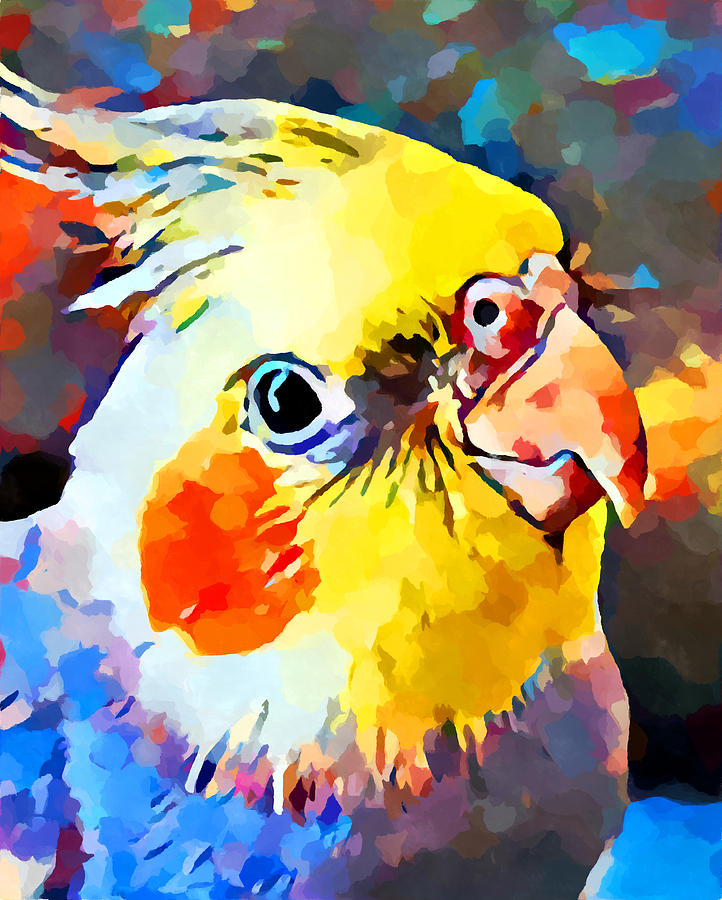This image is a vibrant, detailed watercolor-style painting, possibly created digitally, showcasing a parakeet. The bird, with its bright yellow face and white facial sides, features prominent red circles on its cheeks and a slightly reddish beak. It gazes directly at the viewer, with a posed crest of feathers atop its head. From the face and neck downwards, its feathers transition through shades of blue, deep purple, and bluish gray, dotted intermittently with red. The background complements the bird's eclectic color palette, blending splotches of blue, black, yellow, orange, and grayish blue tones, creating a harmonious and colorful artistic composition.